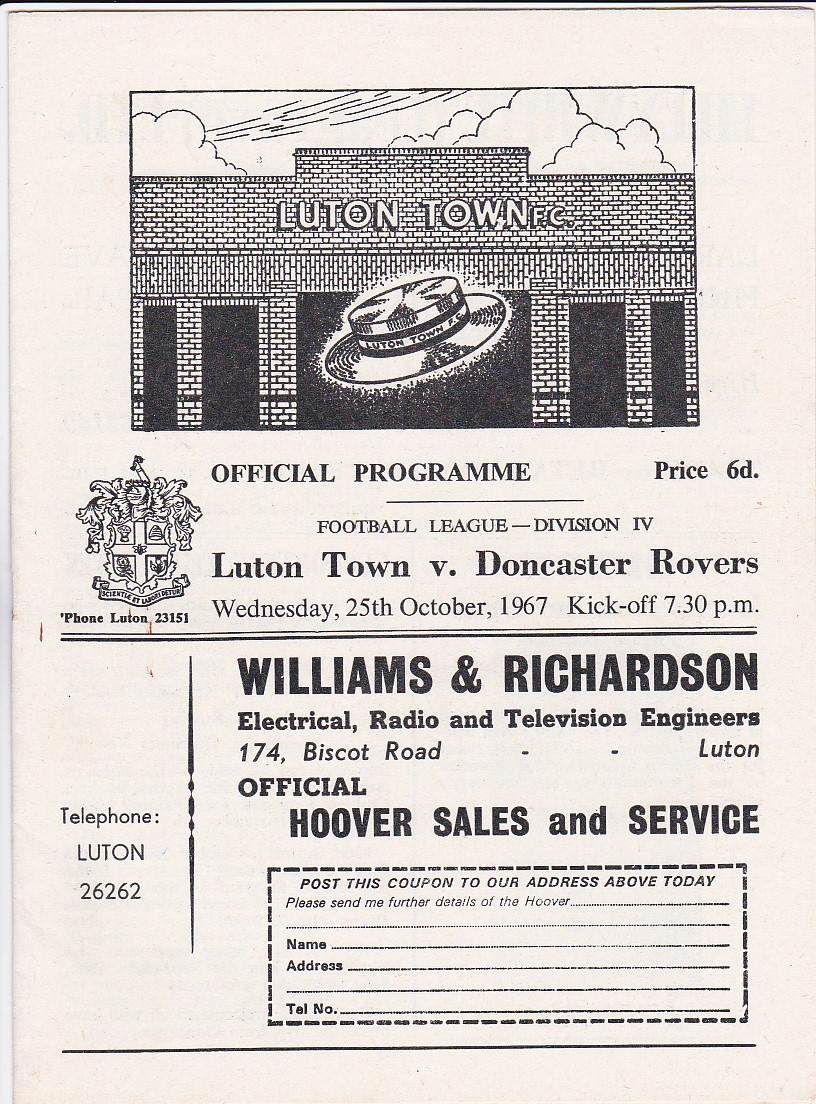The image is a detailed scan of an official program for the Football League Division IV match between Luton Town and Doncaster Rovers, held on Wednesday, 25th October 1967, with a kickoff at 7:30 p.m. At the top, there is a distinctive black-and-white line drawing of a brick building, adorned with long rectangular windows and the text "LUTON TOWN FC" prominently displayed across the top. Hovering above the building is a whimsical hat featuring the same text along its cylindrical portion, suggesting a sense of playfulness or celebration. Surrounding this scene are clouds, hinting at a windy day. Below the image, it reads "Official Program" with a listed price of 6D. Further down, the program details the match specifics: "Football League Division 4, Luton Town versus Doncaster Rovers." The bottom section includes an advertisement for "Williams and Richardson Electrical, Radio, and Television Engineers, 174 Biscott Road, Luton," stating they are official Hoover Sales and Service providers, complete with a telephone number, "Luton 26262." Additionally, there's a coupon area inviting people to request more details about Hoover products by providing their name, address, and telephone number. This comprehensive and nostalgic piece of memorabilia captures the essence of 1960s football culture.